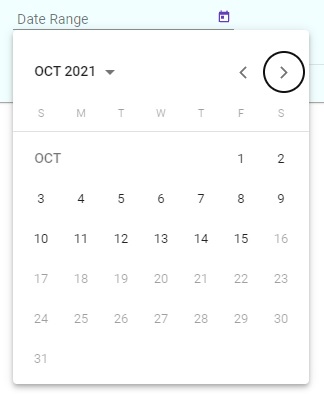A detailed image caption for the screenshot could be:

"This image shows a screenshot of a calendar interface from an app or website. At the top of the calendar, the term 'Date Range' is displayed against a light blue background. To the right of this term, there is a small purple calendar icon. The main calendar is expanded in a white pop-up window, with a drop-down menu at the top left indicating the month 'October 2021.' To the right of this drop-down, there are forward and back arrow icons for navigation, with the forward arrow circled in black. Below these controls, the days of the week are abbreviated as 'S, M, T, W, T, F, S,' with a horizontal line beneath them. The dates of the month are organized in a grid format, starting with the 1st of October on the first Friday and ending with the 31st on the last Sunday."